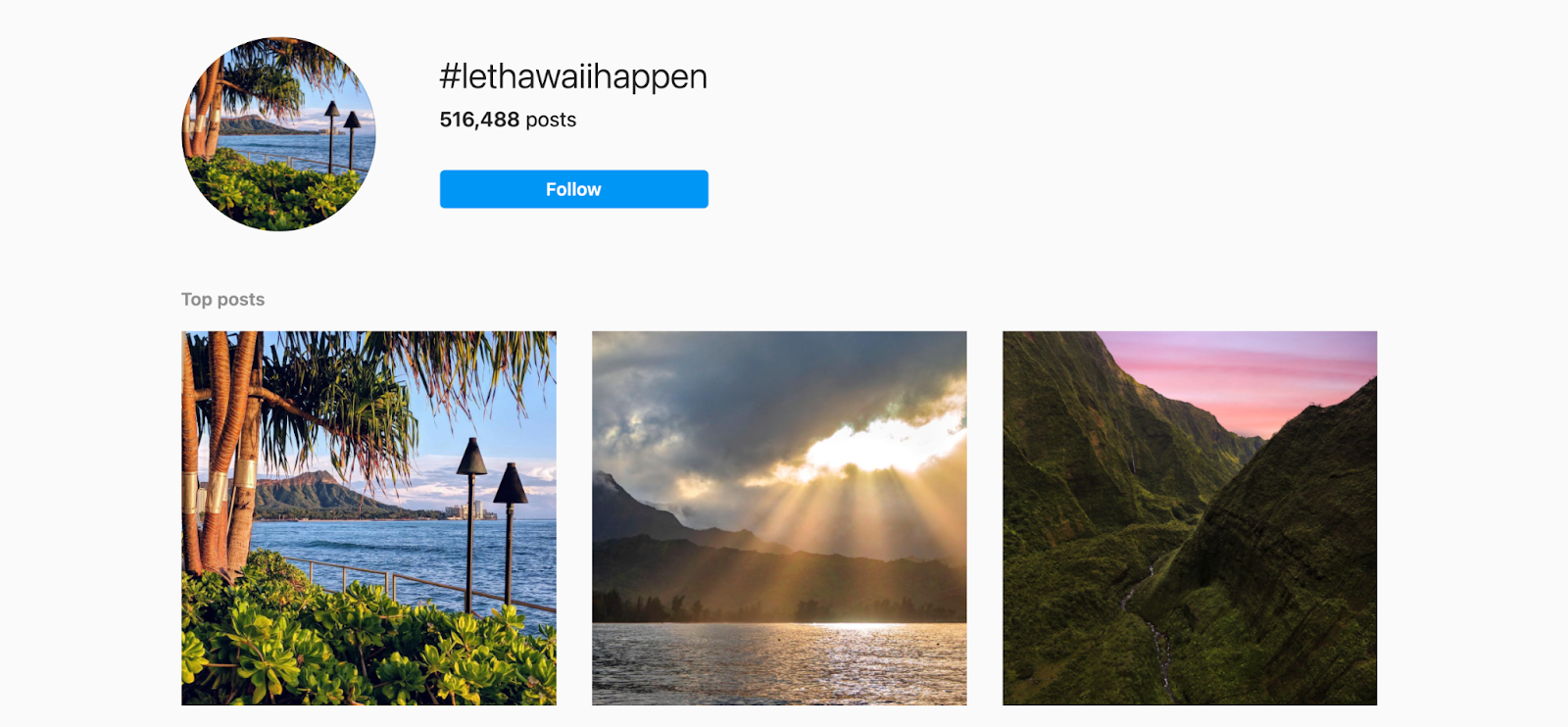A screengrab of a tropical-themed social media post with the hashtag "#lethal" prominently displayed, indicating it has accumulated over 516,488 posts. The top left corner of the image features a stunning profile picture depicting a serene Hawaiian setting, complete with lush vegetation, towering palm trees, and calm waters framed by distant hills. This picturesque scene also includes two tiki bar-style lamps that add to its exotic ambiance. 

Beneath this, the user has shared three additional images:
1. A larger version of their profile picture, showcasing the same tranquil Hawaiian landscape.
2. A similar tropical scene, but this time under a dramatically different sky. Dark, ominous clouds loom overhead, creating a stark contrast with the brilliant rays of sunlight piercing through and reflecting off the water, adding a magical touch.
3. A close-up, artistic shot of a mountain valley. The image captures two steep, dark brown cliffs flanking a narrow valley, with a breathtaking pink sky streaked with white above, likely depicting a mesmerizing sunset or sunrise.

Each photo beautifully captures different facets of nature's splendor in a vibrant tropical setting.